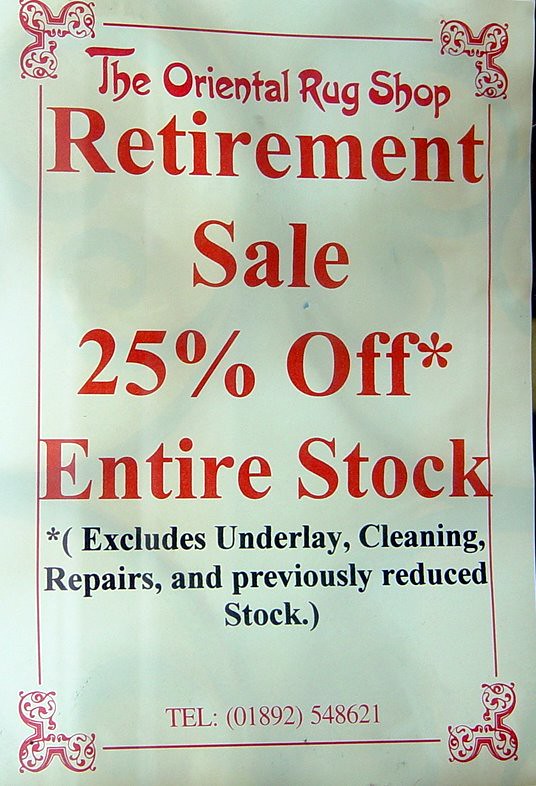This is an advertisement poster for the Oriental Rug Shop Retirement Sale printed on a plain white sheet of paper with hints of blue or green. The poster features a vertical design with a thin red border running along all four edges, comprising intricate designs in each corner, resembling three interconnected circles similar to a three-leaf clover without stems, adorned with squiggly leaf-like patterns inside. The main text, all in red, prominently announces "The Oriental Rug Shop," "Retirement Sale," "25% Off," and "Entire Stock" with an asterisk. Below this, in smaller black text, the asterisk is explained in parentheses: "Excludes underlay, cleaning, repairs, and previously reduced stock." At the bottom of the poster, the contact information is provided in red text: "TEL: (01892) 548621."